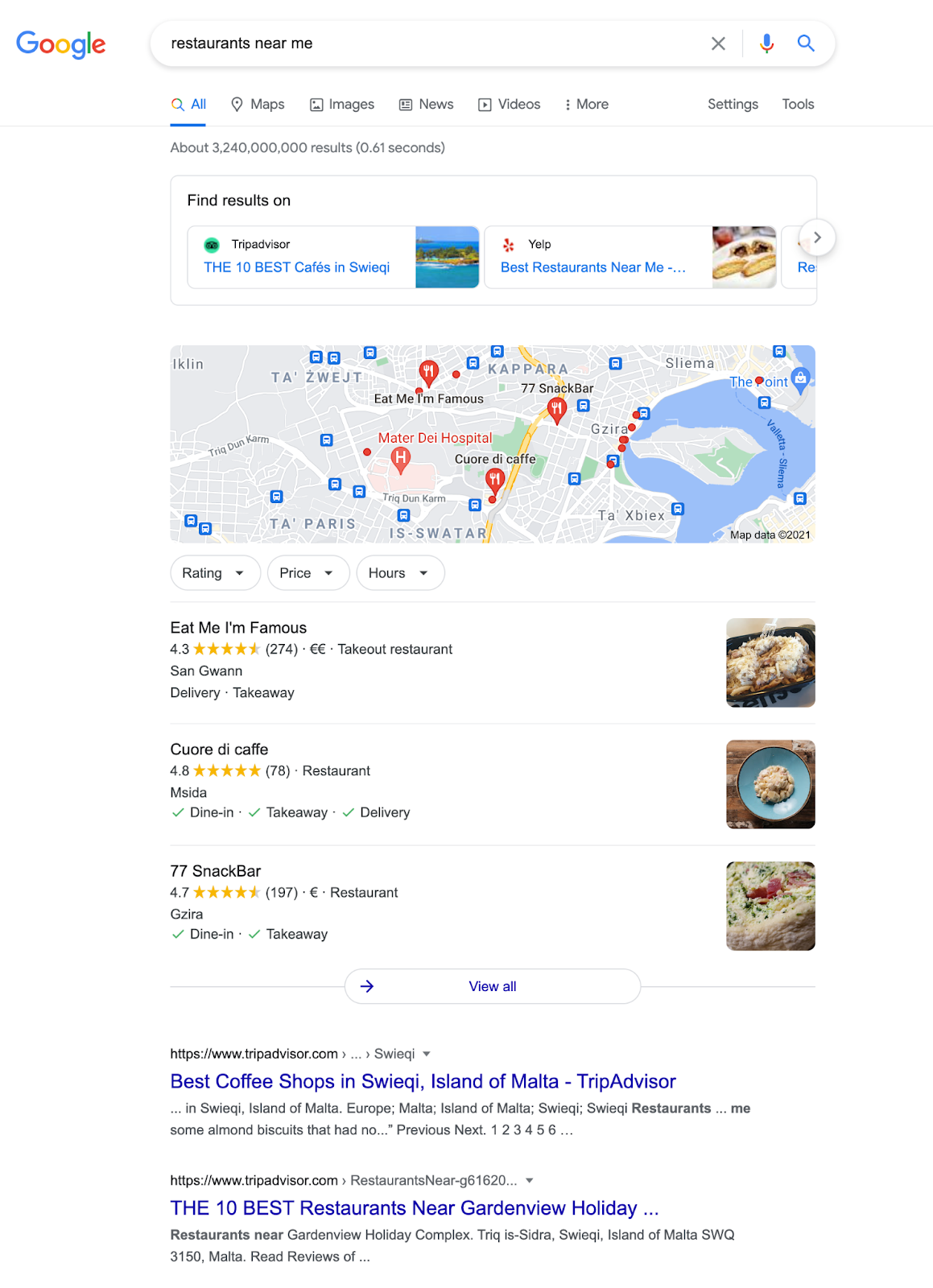The image depicts a Google search results page for "restaurants near me," showing a vast number of results—approximately 3.24 billion—in just 0.61 seconds. The user has clicked on the "All" tab. The search results include several components:

1. **Top Section**:
    - **TripAdvisor Result**: "Find results on TripAdvisor: The 10 best cafes in Swiggy," accompanied by an image of a scenic landscape featuring the sky, the sea, and trees.
    - **Yelp Result**: "Best restaurants near me," with a picture of food on a plate.
    - **Scrollable Section**: Allows users to scroll sideways for more options.

2. **Map Section**: 
    - **Martyr Day Hospital** is centrally located on the map, with several other pins indicating restaurant locations.
    - **Highlighted Restaurants**:
        - **Eat Me I'm Famous**: 4.3 stars, 274 reviews. Described as a takeout restaurant located in San Juan. Offers delivery and takeaway. An accompanying image shows food.
        - **Kwanda Cafe**: 4.8 stars, 78 reviews. Offers dine-in, takeaway, and delivery. The image features a blue plate of food.
        - **Snack Bar 77**: 4.7 stars, 197 reviews. A restaurant symbolized by a single euro (€), indicating price range. Offers dine-in and takeaway, with a close-up image of various colored foods (white, red, green).

3. **Additional Results**:
    - **TripAdvisor Result**: "Best coffee shops in Swiggy, Island of Malta," followed by text.
    - **Other Listings**: "10 best restaurants near Garden View Holiday Complex, Swiggy, Isle of Malta."

The detailed layout indicates various filters, including rating, price, and hours, making it easier for users to find specific types of dining options.